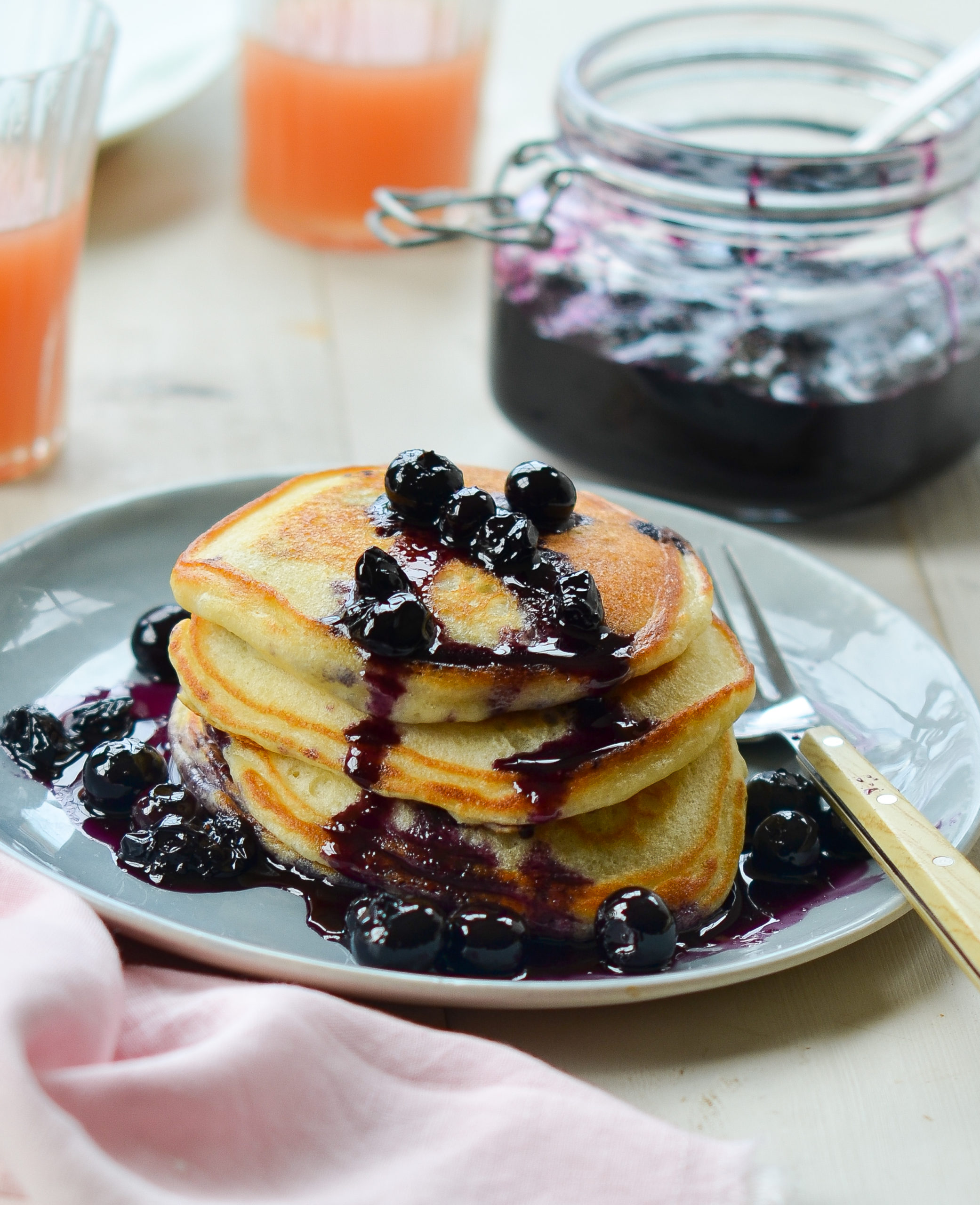This photograph captures a delightful breakfast setup, centered around a porcelain plate of pale blue color displaying a stack of golden, brownish-yellow pancakes. The pancakes are topped with dark navy-blue blueberries and a rich, dark blue blueberry syrup that cascades down their sides. Positioned next to the stack is a silver fork, reflecting the morning light. Adjacent to the plate on the right side, a glass jar brimming with what appears to be homemade blueberry jam, complete with visible chunks of blueberries and a spoon resting inside, further enhances the inviting scene. The breakfast ensemble rests on a pink fabric laid across a nearly white wooden table. Adding a refreshing touch, two partially filled glass containers of orange juice complete the picturesque morning meal. This image not only emphasizes the warm, toasty appeal of the pancakes but also harmoniously presents the surrounding elements, making it mouthwateringly inviting.